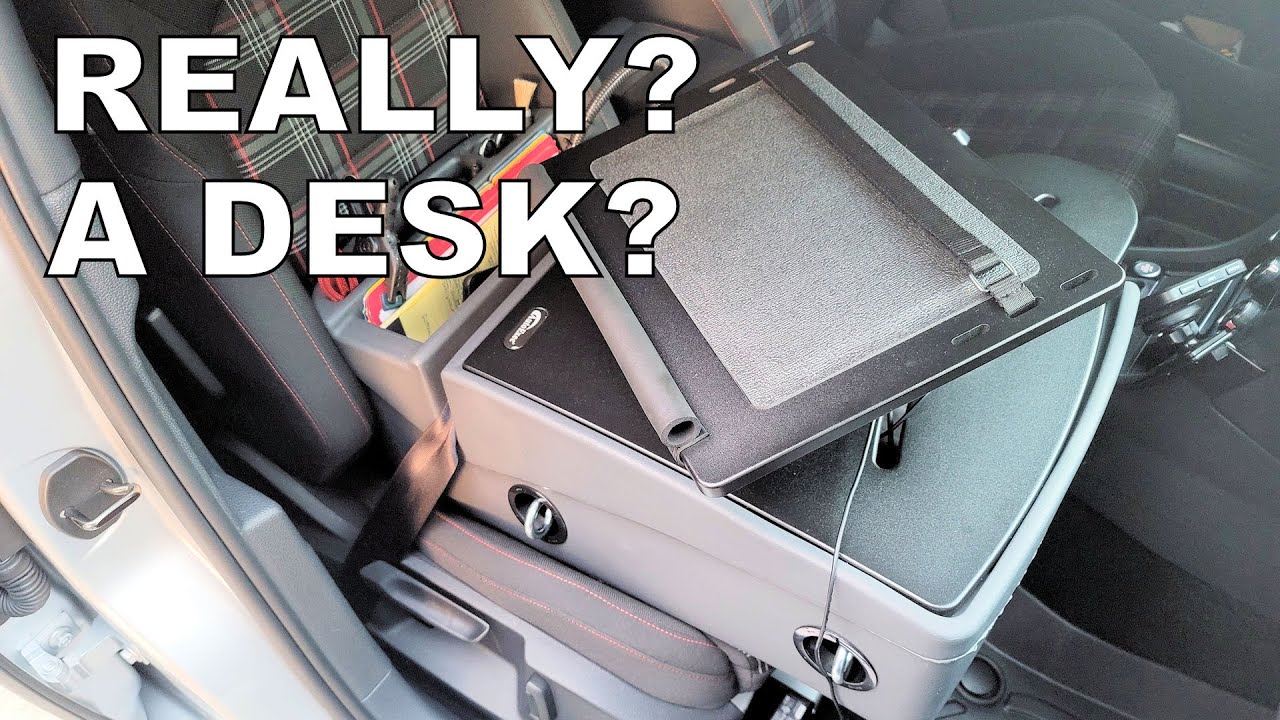The image depicts the interior of a gray car, focusing on the front passenger seat. The seat features a checkered plaid pattern in black, gray, and red lines. Central to the image, a black desk or tray is securely seat-belted to the front passenger seat, functioning as an unusual makeshift desk with a strap running horizontally across it. The seat's back also boasts a plaid design, contrasting with the overall gray interior, including the seats, floor, and door jams. A silver circle and handle are visible at the bottom left. At the upper left-hand corner, large white sans-serif text exclaims, "Really? A Desk?" highlighting the unconventional use of the seat as a workspace.